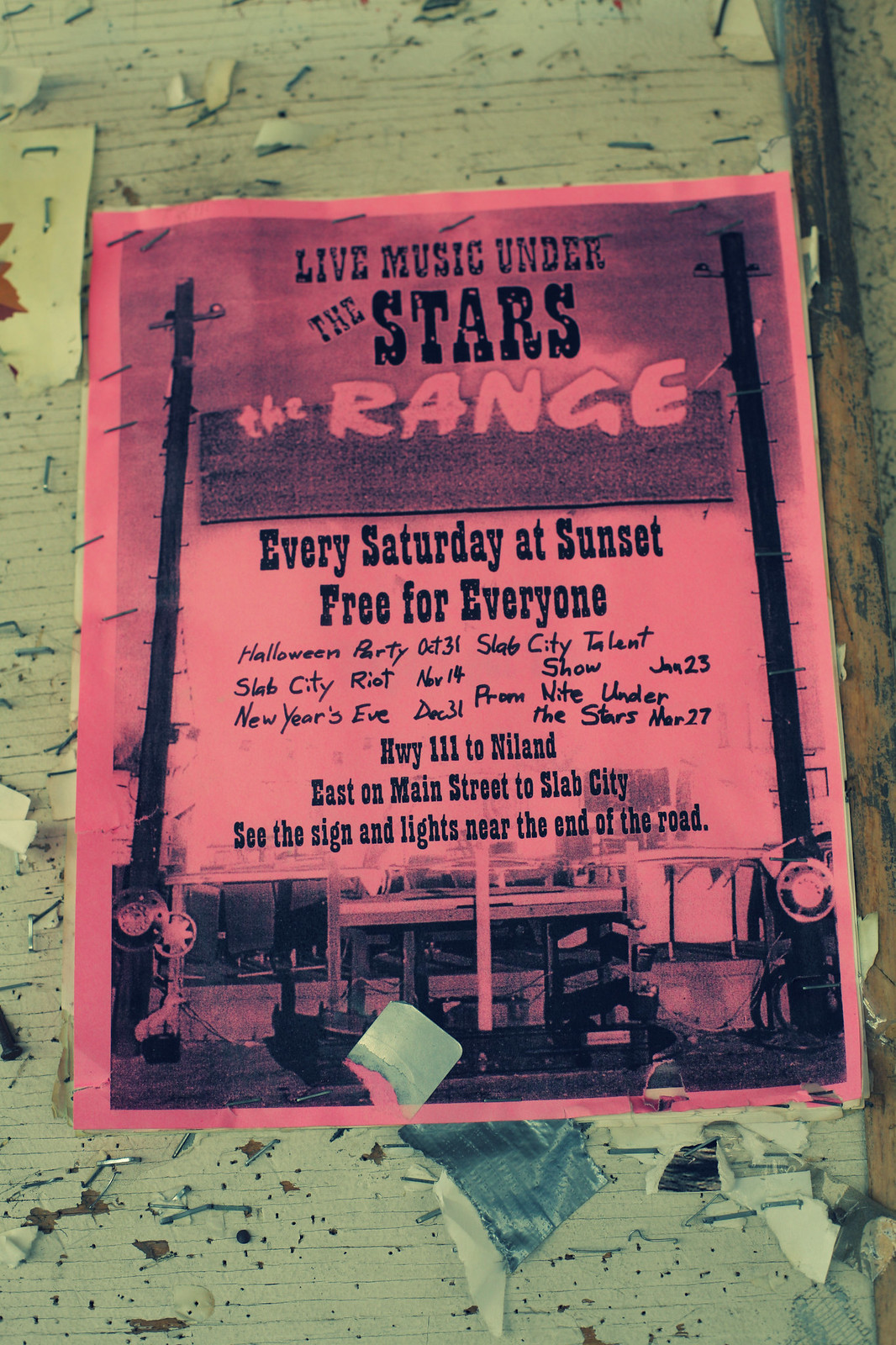This photograph captures a promotional poster for a live music event, prominently displayed on a white, somewhat damaged wall. The rectangular poster is a vivid pink and is secured using multiple metallic pins and staples, which are scattered around the edges, indicating it has been placed amidst other advertisements in the past. The primary text reads: "Live Music Under the Stars at The Range." Beneath this heading, it proclaims: "Every Saturday at sunset, free for everyone."

Further details are inscribed below, including several event dates and descriptions such as a Halloween Party on October 31st, Slab City Talent Show on November 14th, New Year's Eve event on December 13th, and a Prom Night Under the Stars on March 27th. There is additional handwritten text providing directions: "Highway 111 to Niland, east on Main Street to Slab City. See the signs and lights near the end of the road." 

The poster is notably dark pink with black text and has an image at the bottom, potentially depicting an exterior view related to the event locations. Overall, this highly detailed and colorful poster is a vibrant call to a series of musical gatherings.